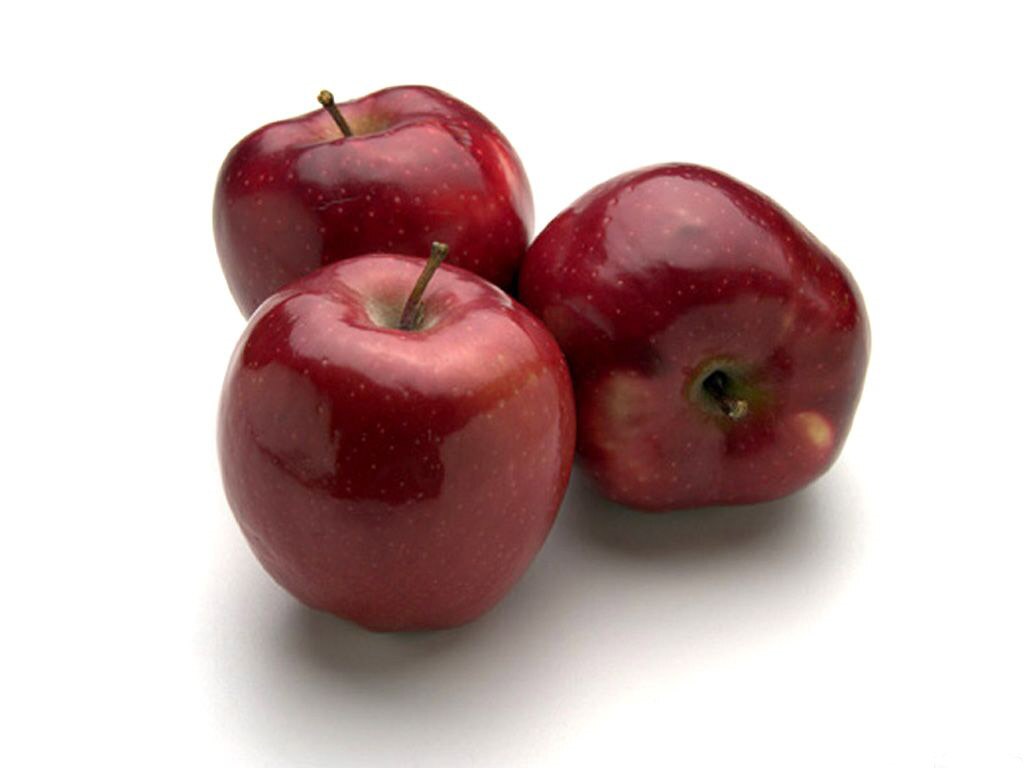The image features three deep red apples with a glossy, reflective texture, resting on a white tabletop that contrasts sharply with their rich color. They cast faint, grayish-tan shadows beneath them, adding depth to the scene. The apples, each with a brown stem, exhibit small yellow speckles, reminiscent of tiny pricks from a toothpick.

In the foreground, one apple stands upright, its stem facing upward. Directly behind it, a second apple also stands upright, but its stem points in the opposite direction, making it appear slightly duller due to the light's angle. To the right, an apple lies on its side with its stem facing forward, presenting an interesting, misshapen form. This arrangement of apples creates a visually appealing composition, emphasizing their varying orientations and the interplay of light and shadow on their polished surfaces.